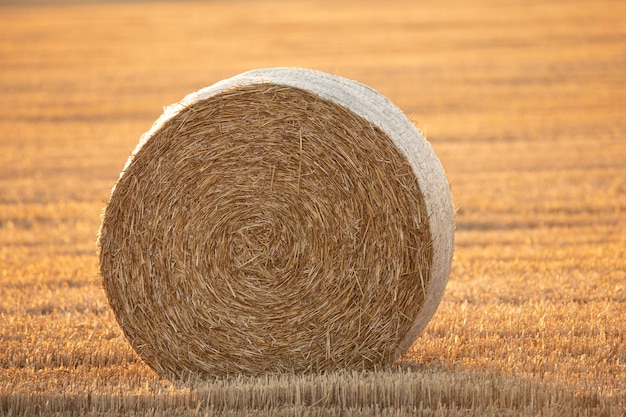In this serene, early morning or late midday landscape, a large, tightly wound cylindrical hay bale stands prominently in the foreground of a recently harvested field. The field’s hues of brown, gold, and tan stretch out to the horizon, emphasizing the freshly cut wheat that forms a muted but cohesive backdrop. Close to the hay bale, individual stalks protrude slightly higher than those in the distance, creating a subtle gradation in height. The sun, while not visible in the image, casts a gentle glow, contributing to the peaceful ambiance and casting soft shadows around the bale. This meticulously rolled cylinder of dried wheat, held together with a film around its edge, displays precise, concentric circles of tightly packed hay, adding a textural detail to the overall calm and quiet of the rural scene.